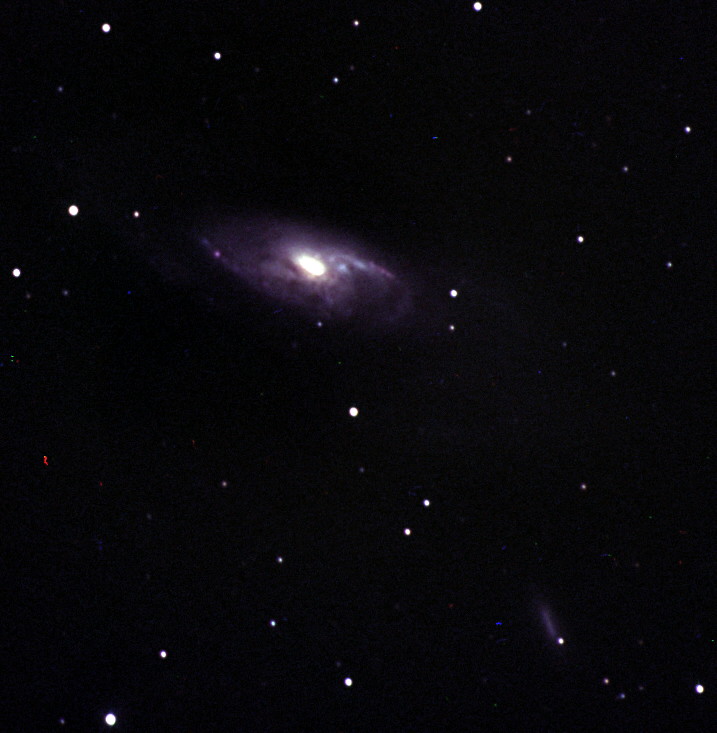This photograph taken from space features a black, star-studded background with numerous white stars scattered across the image, along with a small red star situated on the middle-left side. Dominating the upper center of the image, just slightly off to the left, is a significant bright white star encircled by a luminous haze with a subtle purplish hue, creating a glowing effect that seems to illuminate the area around it. This central star appears to be surrounded by spiraling clouds, adding an intricate and mesmerizing quality to the scene. Notably, in the bottom left corner, one star seems to be moving within the frame. The photograph is devoid of any text or dates, emphasizing the natural, undisturbed beauty of outer space.